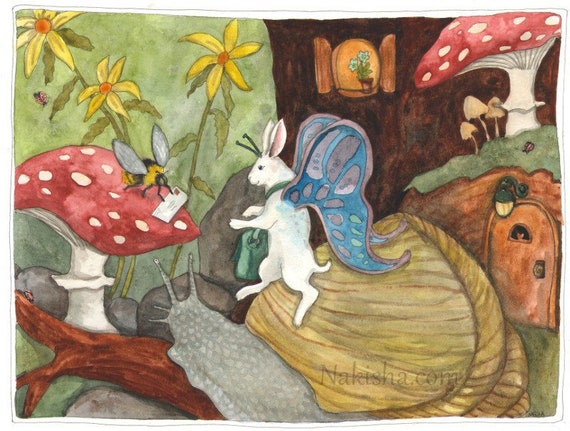This horizontal rectangular image appears to be a vibrant children's drawing imbued with whimsical details. At the center of the scene stands a rabbit-like creature with bluish wings, placed on a sturdy wooden platform. Its upright ears and playful expression enhance its animated appearance. The rabbit seems to be engaged in conversation with a bug perched atop a toadstool that features a white stem and a red cap adorned with white dots. A large gray bug, with only its back visible, stands closely next to the rabbit, adding to the scene's curious allure.

The background, reminiscent of a lush garden, is painted green with sprouting yellow flowers, giving the impression of grass and a flourishing environment. Toward the right side of the image lies another toadstool, beneath which grow several small brown toadstools, creating a layered mushroom habitat. Below this, a quaint door leads into what seems to be a hidden cabin, notable for inviting a yellow glow, suggesting warmth and shelter within. Above the rabbit's majestic wings, a small window is nestled into the scenery, contributing an element of domestic coziness to this enchanting garden tableau.